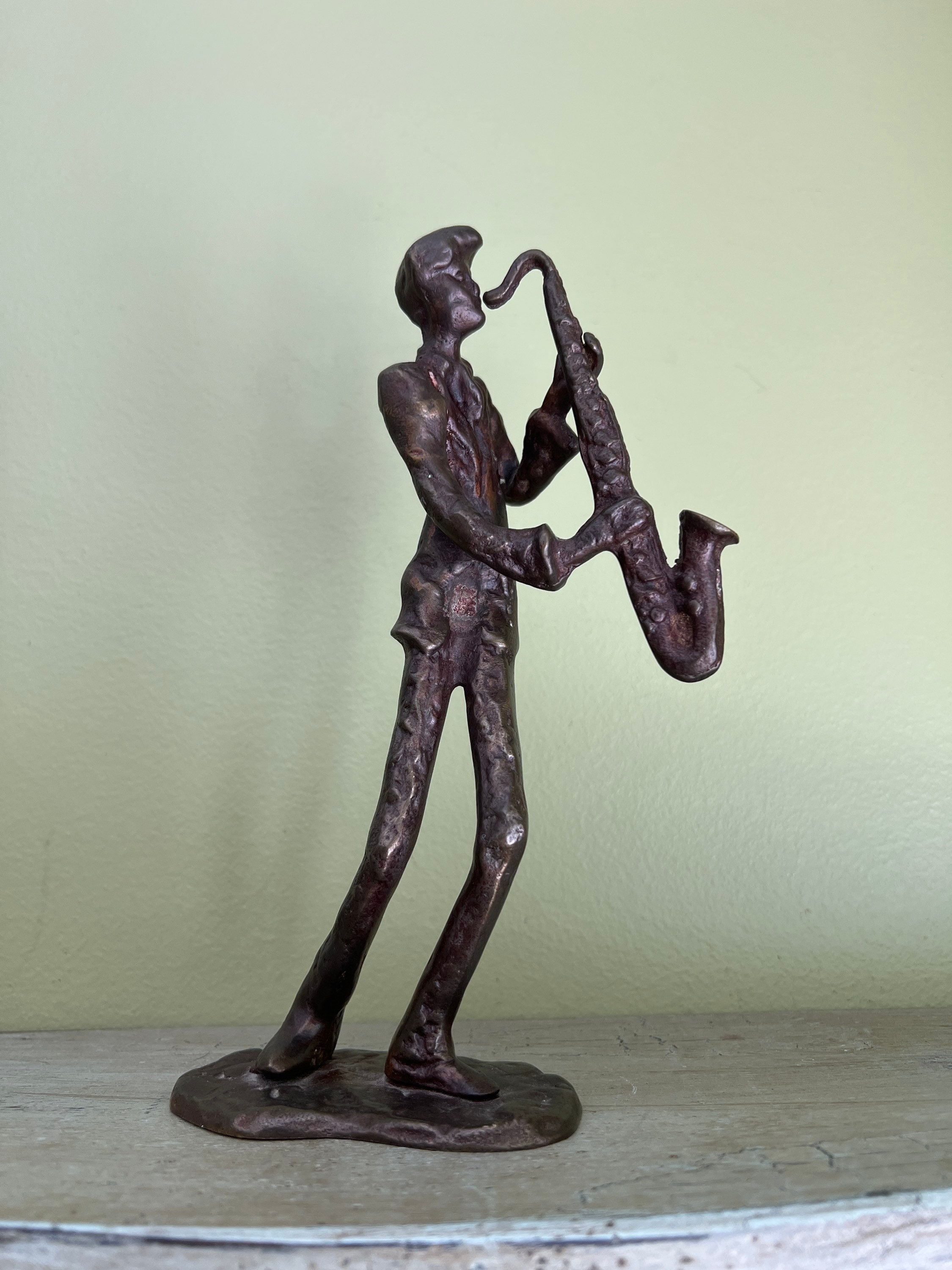This photograph features a detailed bronze statue with an unpolished finish depicting a slender, modernistic man intensely playing a very long saxophone, which almost matches his height. The artist exaggerated the man's lanky proportions, giving him exceptionally long arms and hands, which enhances the visual harmony with the extended saxophone. He appears to be leaning dramatically into the saxophone, adding a sense of movement and dedication to his performance. The statue is adorned in attire reminiscent of the 1960s or early 70s, including bell-bottom pants, a jacket with bulging pockets, and a pompadour hairstyle, similar to an Elvis or 1950s bouffant style. The statue stands on an oval-shaped brown base placed on what appears to be a wooden surface or shelf. The background showcases a wall painted in a muted light green, adding a subtle contrast to the dark brown metal of the statue.